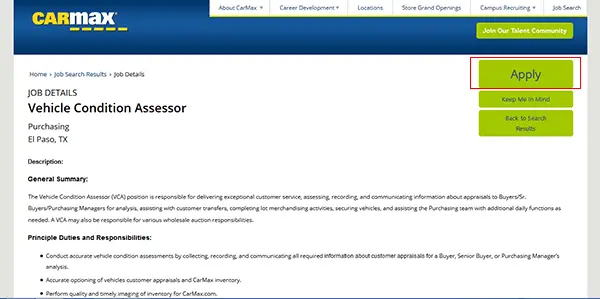**Screenshot Description:**

The screenshot features a bright white background with the CarMax logo prominently displayed. The "Car" part of the logo is colored yellow, while "Max" is in white, standing out clearly against the backdrop. The screenshot captures an interface showing home job search results and specific job details.

**Job Title:**
Vehicle Condition Assessor (VCA)

**Location:**
El Paso, Texas (TX)

**Job Description:**
- **General Summary:** The Vehicle Condition Assessor (VCA) role is integral to delivering exceptional customer service. 
- **Responsibilities:** 
  - Assessing, recording, and communicating detailed information about vehicle appraisals to buyers, including Senior Buyers and Purchasing Managers, for further analysis.
  - Assisting with unspecified computer-related tasks.
  - Managing lot merchandising activities, ensuring the proper security of vehicles, and evaluating vehicles to assist with purchasing decisions.

The job listing appears to be hosted by CarMax and specifically targets potential candidates in El Paso, Texas. The description emphasizes the importance of customer service and attention to detail in the assessment and recording processes.